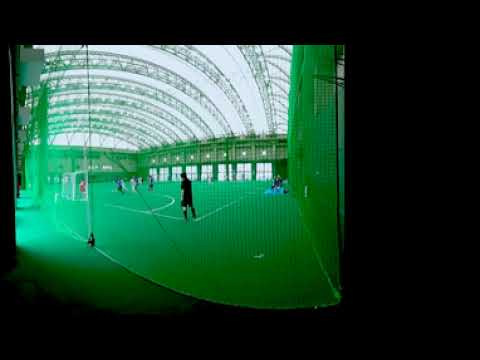The photograph captures an indoor soccer field bordered by green walls and netting. The field appears to be covered with astroturf rather than natural grass. A distinct domed or retractable ceiling allows generous natural light to flood the scene. White lines mark the boundaries, including a clearly defined goalie box. There is a soccer goal on the left side of the image, where the goalie, dressed in a red shirt, is positioned. In the center foreground, a player outfitted in black shirt, shorts, and socks stands prominently. To the right corner of the field, another player in black attire is visible, with green walls matching the field in the background. Despite the somewhat darker periphery, the middle area is well illuminated, highlighting the players involved in the game.